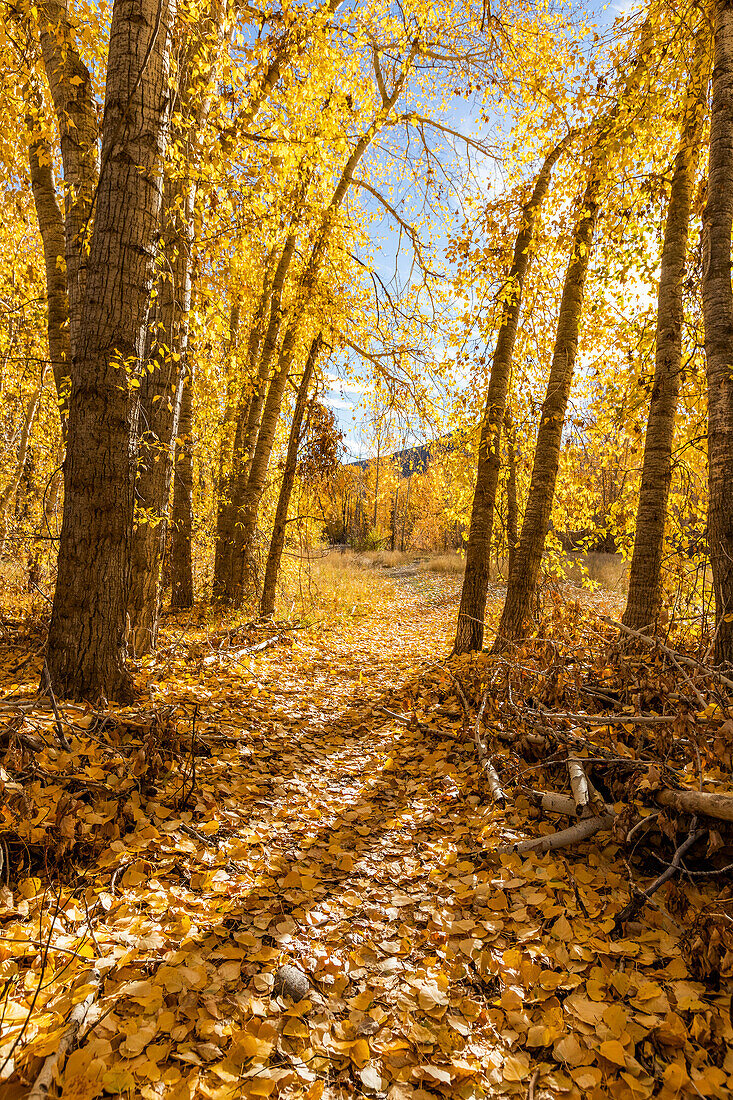This vibrant fall scene captures the enchanting essence of autumn. The photograph, taken outdoors during fall, showcases a wooded forest adorned with tall trees predominantly exhibiting golden yellow and orange leaves. Strewn across the ground, these colorful leaves create a thick carpet, nearly obscuring the grass beneath. To the right side of the image, there is a noticeable pile of branches and limbs, with similarly hued leaves attached to them. On the left, more branches and clusters of trees are visible.

A path meanders through the forest, flanked by trees on both sides, inviting the viewer deeper into the woods. Farther along this path, additional trees with golden foliage continue to pepper the landscape. The sky overhead is a clear blue, with a few wispy white clouds. In the distance, there's a hint of a brown-roofed building or perhaps a mountain range, adding depth to the scene. Shadows cast by some of the trees stretch towards the foreground, enhancing the texture and contrast within the image. This snapshot beautifully encapsulates the serene and picturesque beauty of fall.